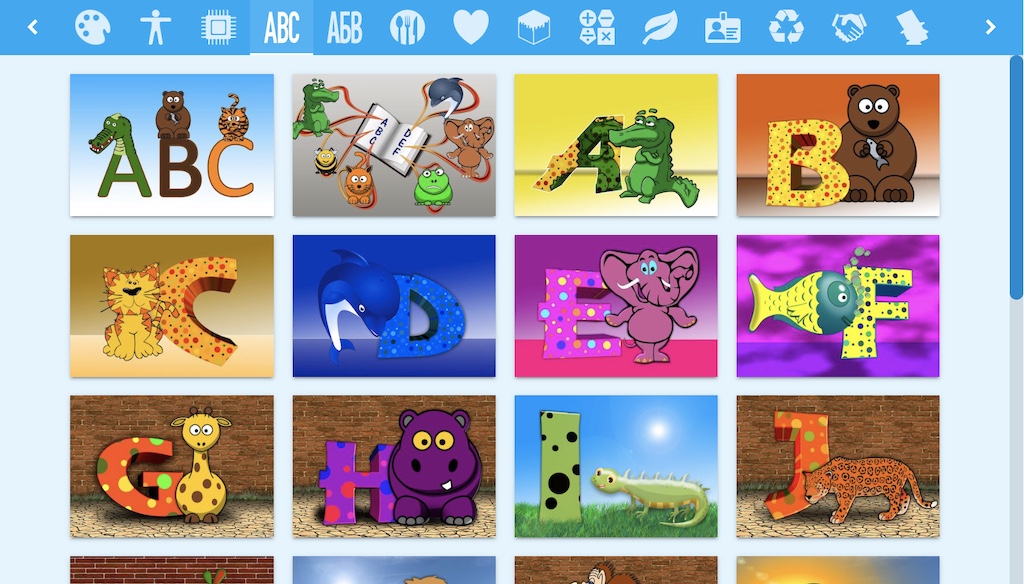The image depicts an online learning activity designed to teach children the alphabet. The website features a prominent blue bar at the top, crowded with various icons representing different categories such as art, people, ABCs, food, hearts, geometric shapes, math, leaves, and recycling, among others.

Beneath the navigation bar, the main content is organized into multiple rows of squares. Each square contains an alphabet letter paired with an animal illustration. In the topmost row, starting from the left, the first square displays an 'A' with an alligator, a 'B' with a bear, and a 'C' with a cat perched on top of it. To the right of this, a square displays a book titled "ABCDEF" with animals pointing towards different letters.

The second row showcases the letters and their corresponding animals in individual squares: 'A' with an alligator, 'B' with a bear, 'C' with a cat, 'D' with a dolphin, 'E' with an elephant, and 'F' with a fish. Continuing downward, the third row presents 'G' with a giraffe, 'H' with a hippo, 'I' with a small animal that appears to be a lizard, and 'J' with a jaguar.

On the right side of the screen, a vertical blue scrollbar indicates that the page continues further down, offering more alphabet squares that are not currently visible in the image.